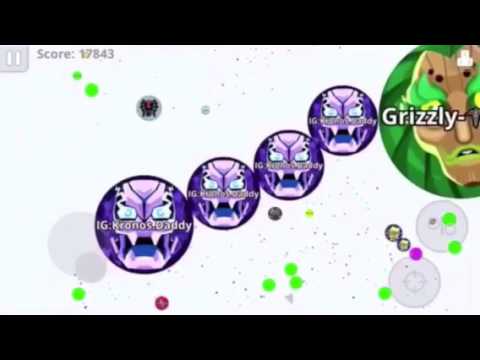The image is a wide rectangular screenshot of a video game, bordered by thick black strips at the top and bottom. The background is an off-white or light gray color scattered with neon green, purple, and gold dots. In the center, there are four purple circular objects featuring a design that resembles an angry purple robot or monster face with blue, glowing eyes, and sharp fangs. Each of these circles has the text "IGKRANOSDADDY" on them. 

In the top right corner, there's a larger green circle displaying a man's face with green eyebrows and the name "GRIZZLYDASH" beside it. This face appears somewhat eerie due to its glowing neon green elements. On the top left corner of the screen, a gray pause button is visible along with a score of 17,843.